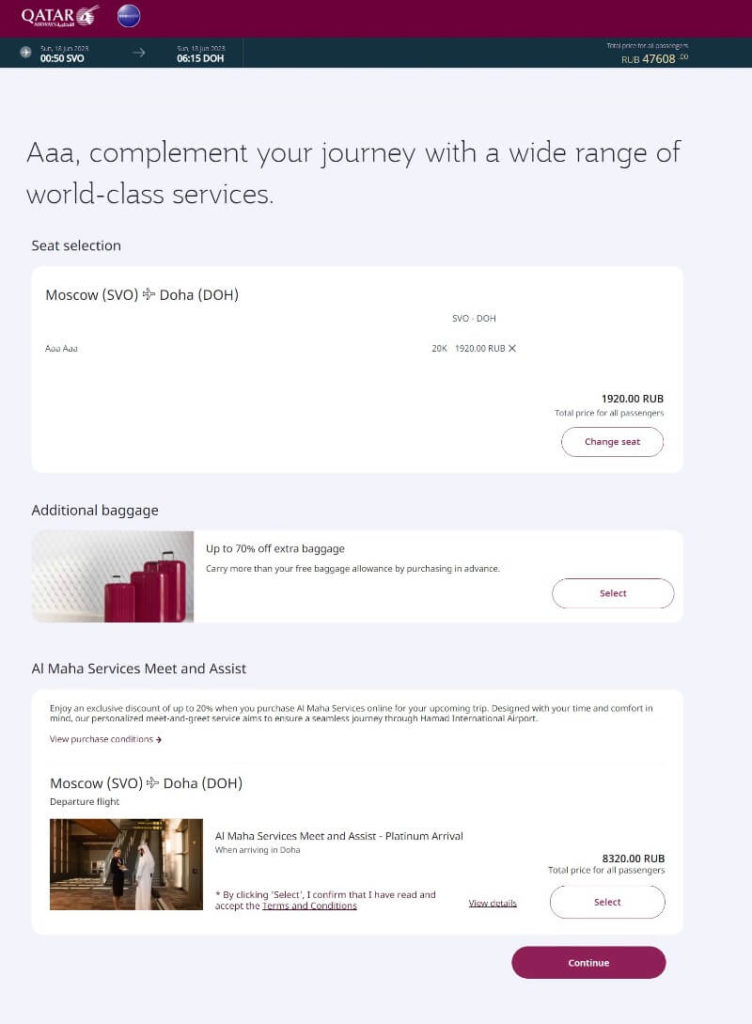"Screenshot of Qatar Airways' website featuring travel options. The maroon header at the top displays the 'Qatar Airways' logo in white. Beneath it, a dark grey navigation bar provides additional options. On the left side of the main content area, details of a flight from Moscow to Doha are shown, with the price listed on the far right in RLB. Below the flight information, the website offers an invitation to 'Complement your journey with a wide range of world-class services' and highlights the seat selection feature. A prominent pill-shaped 'Select Seat' button is visible, enhancing user interaction."